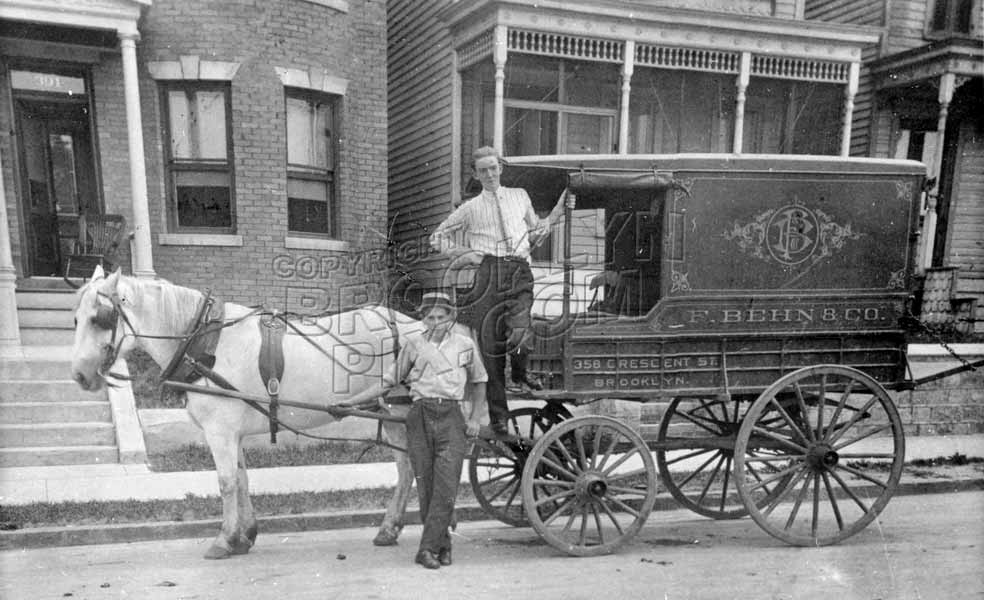This rectangular, black-and-white landscape photograph captures a nostalgic scene from an era before motor vehicles. In the foreground stands an antique black buggy harnessed to a white horse, facing left. Two men are positioned near the horse, one holding the reins with a cigarette dangling from his mouth, sleeves rolled up, and donned in baggy trousers and shoes. The other man stands beside the carriage, his white dress shirt buttoned down, also wearing trousers and shoes. Both men are dressed in early 20th-century attire. The side of the stagecoach bears the inscription "358 Crescent Street, Brooklyn, New York" along with the logo "F.BEHN & CO." The background features a row of three townhomes; the leftmost is constructed of brick, while the other two appear to be wooden. Steps descend from the brick house to the sidewalk below. Overlaying the image is a clear text watermark that reads "copyright brooklynpics.com." The scene evokes a sense of history, depicting a time when life was slower and horse-drawn carriages were a common sight.